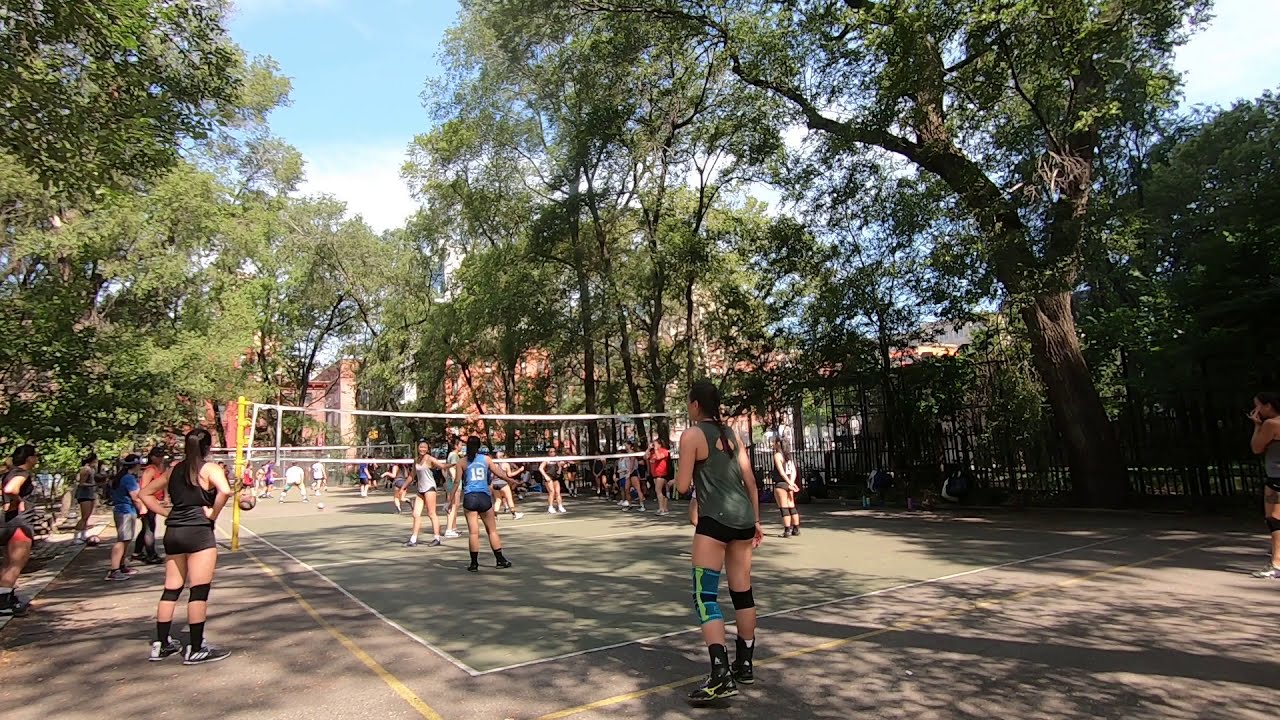In the foreground, several women are engaged in an outdoor volleyball game on a light green court surrounded by a dark concrete boundary. The net stands prominently in the middle, and the court is dappled in shade from towering trees, some reaching about 30 feet in height, their sprawling branches casting shadows across the players. The sky overhead transitions from a vibrant turquoise to a pale white haze, dotted with a few clouds but mostly clear, indicating a sunny day.

Closest to the camera, a player wearing a dark top and sporting a blue and green knee brace on her left knee is poised to join the action. In front of her, another player dons a light blue shirt emblazoned with the number 19 on the back. Scanning the scene, numerous women, all in various athletic outfits—some in sleeveless shirts of gray and blue hues, others in short shorts or knee-length shorts, many with knee pads or braces—are scattered both on the court and along the sidelines, either playing or observing.

Set within a park, with one large tree particularly prominent in the right background and more trees forming a leafy barrier around the area, the scene also features a second volleyball court in the background. The entire recreational area is enclosed by a sturdy black metal fence, beyond which a row of tall buildings is distantly visible. The volleyball lies on the ground near the back court, symbolizing a brief pause in the energetic proceedings.